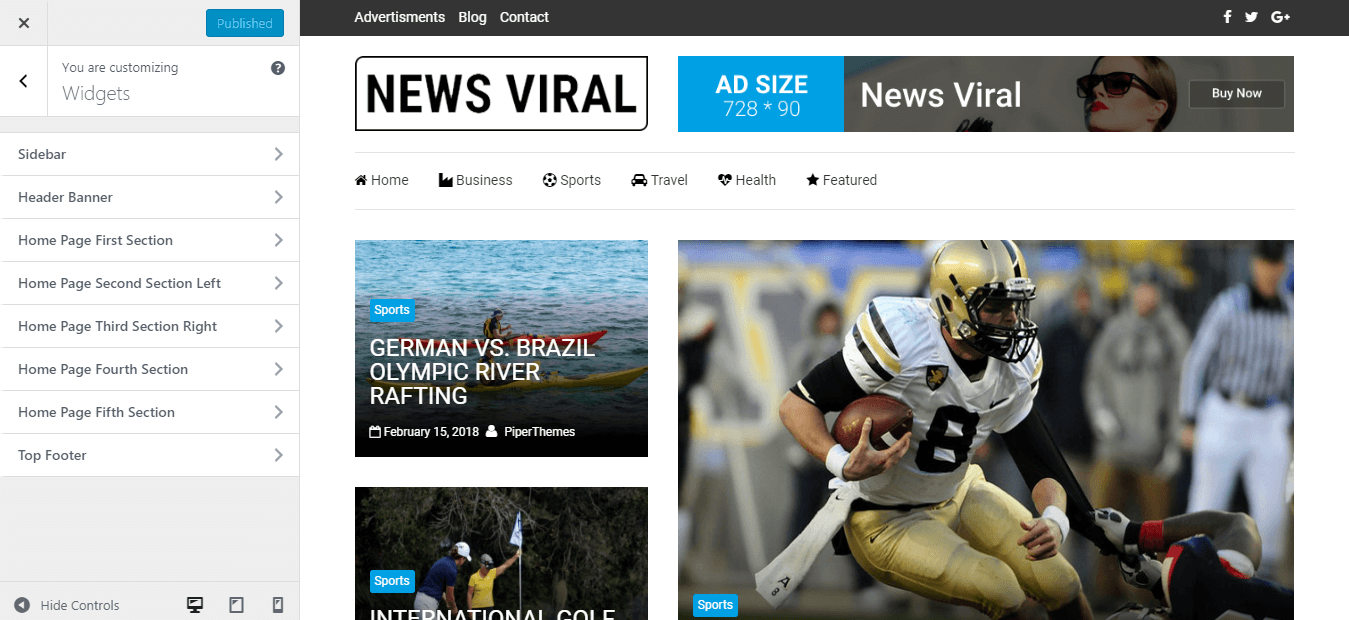This image depicts the interface of a website building platform, specifically showcasing the News Viral section. The top portion of the layout includes an advertising space measuring approximately 728x90 pixels, branded with the News Viral logo. Directly below the ad space, several navigation tabs are visible, labeled "Home," "Business," "Sports," "Travel," "Health," and "Feature," with a highlighted section for "German vs. Brazil."

Further down, the title of an article appears: "Olympic River Rafting International." Some text is obscured, but it is followed by another section seemingly dedicated to "Golf" and "Football" under the Sports category. On the right side of the screen, a sidebar labeled "Hennepin" is present.

The overall view is that of a user interface for customizing a website. The details include adjustable elements such as the homepage, various sections (first, second, left third, right third, fourth, fifth), a top footer, and possibly a sidebar and header/banner adjustments. The interface allows the user to position their advertisements and curate article placements, providing a comprehensive guide for setting up and organizing different components of the webpage.